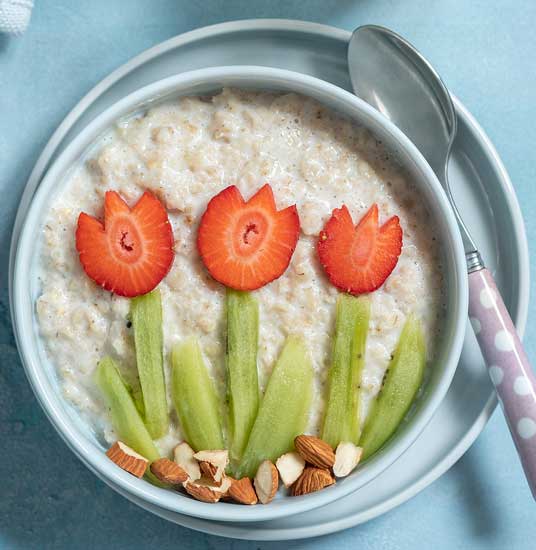This top-down photograph showcases a meticulously arranged bowl of oatmeal, set atop a matching light blue plate on a sea-green table. The oatmeal is garnished with a charming floral arrangement: three strawberries are intricately cut to resemble tulips, complete with stems and leaves fashioned from green kiwi slices. At the base of these fruity 'flowers,' there are chopped almonds simulating soil. A silver spoon with a purple and white polka dot handle rests to the right of the bowl, adding a playful touch to the serene breakfast scene. The oatmeal has a milky consistency, adding to the overall appealing presentation.